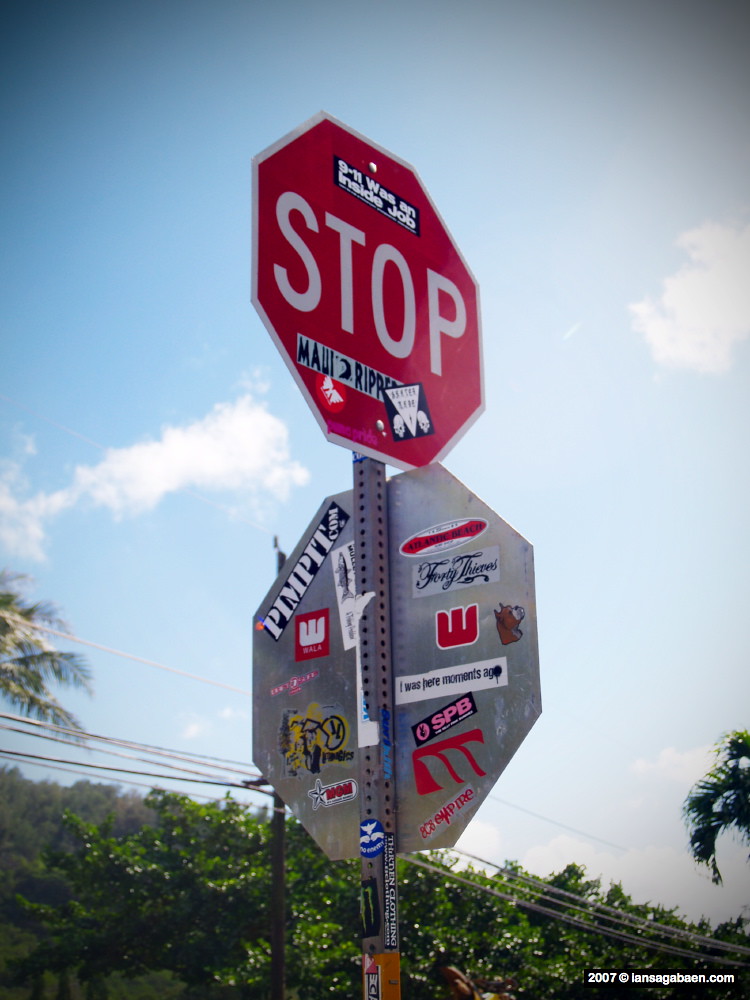The image depicts a pair of hexagonal stop signs outdoors, mounted on a steel rod with vertical holes, situated under a clear blue sky with wispy white clouds. The stop sign facing the camera is red with a white border and the word "STOP" in white letters, featuring several bumper stickers—most notably a black one with "9-11 was an inside job" in white letters, and another saying "Maui Ripper". Additionally, there are a few smaller, illegible stickers. Below this sign, the back of another stop sign is visible, also covered in numerous stickers including one that says "PIMPIT.COM" in black and white, "40 Thieves," "I was here moments ago," and others with mixed red, white, and black designs. Both signs are in a setting with power lines, telephone poles, palm trees, and other foliage in the background. The bottom right corner of the image contains a black text box with "2007, copyright IanSagabayan.com" in white type, indicating the photographer's credit.